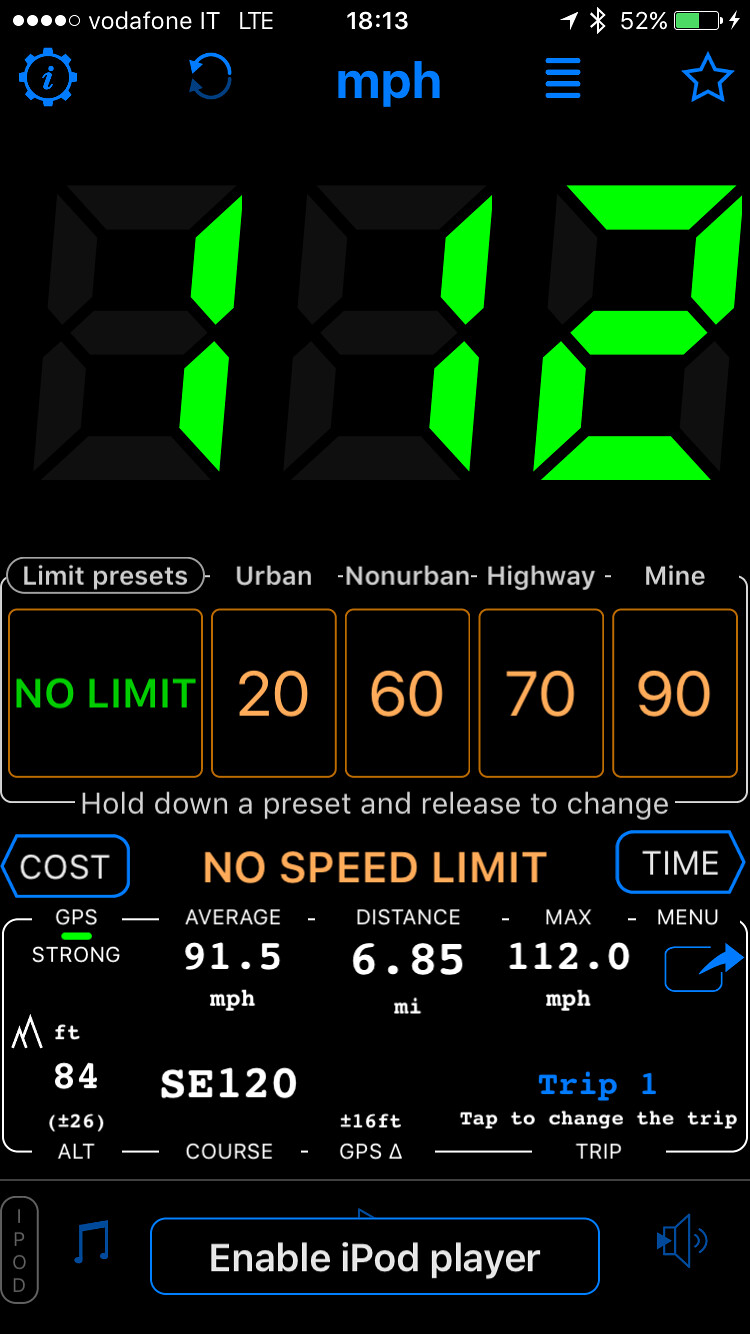The screenshot shows the interface of a speedometer or GPS unit on a phone or iPod, possibly used for a motorcycle. At the top, there are blue icons including a wrench with an eye in it, two blue arrows arcing to the left and meeting at their tips, and a blue acronym, MPH, suggesting speed metrics in miles per hour. 

Next to these icons is a hamburger menu, followed by a star icon. Below them in large green font is a prominent '112'. Underneath this, black boxes with gold outlines display various speed limits: 'No Limit' in green, and '20, 60, 70, 90' in orange.

The bottom section provides detailed trip information in smaller text: 'Average MPH: 91.5', 'Distance: 6.85 miles', and 'Max: 112 MPH', along with indications about direction and trip summaries. The screenshot appears to be a comprehensive display featuring speed metrics, presets, and real-time navigation information.